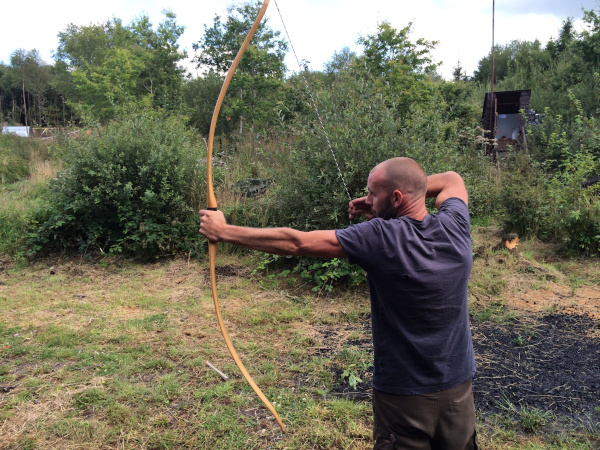The image captures a young man with a shaved head, intensely focused as he prepares to shoot a large bow and arrow in an outdoor setting. He is wearing a light blue, short-sleeved t-shirt and brown pants. The scene is set in a wooded area, evident from the green leaves scattered on the beige ground and the numerous trees in the background. A tent can also be seen in the distance. The young man appears to be practicing archery for therapeutic purposes, showcasing a serious and concentrated demeanor as he draws the bowstring back.